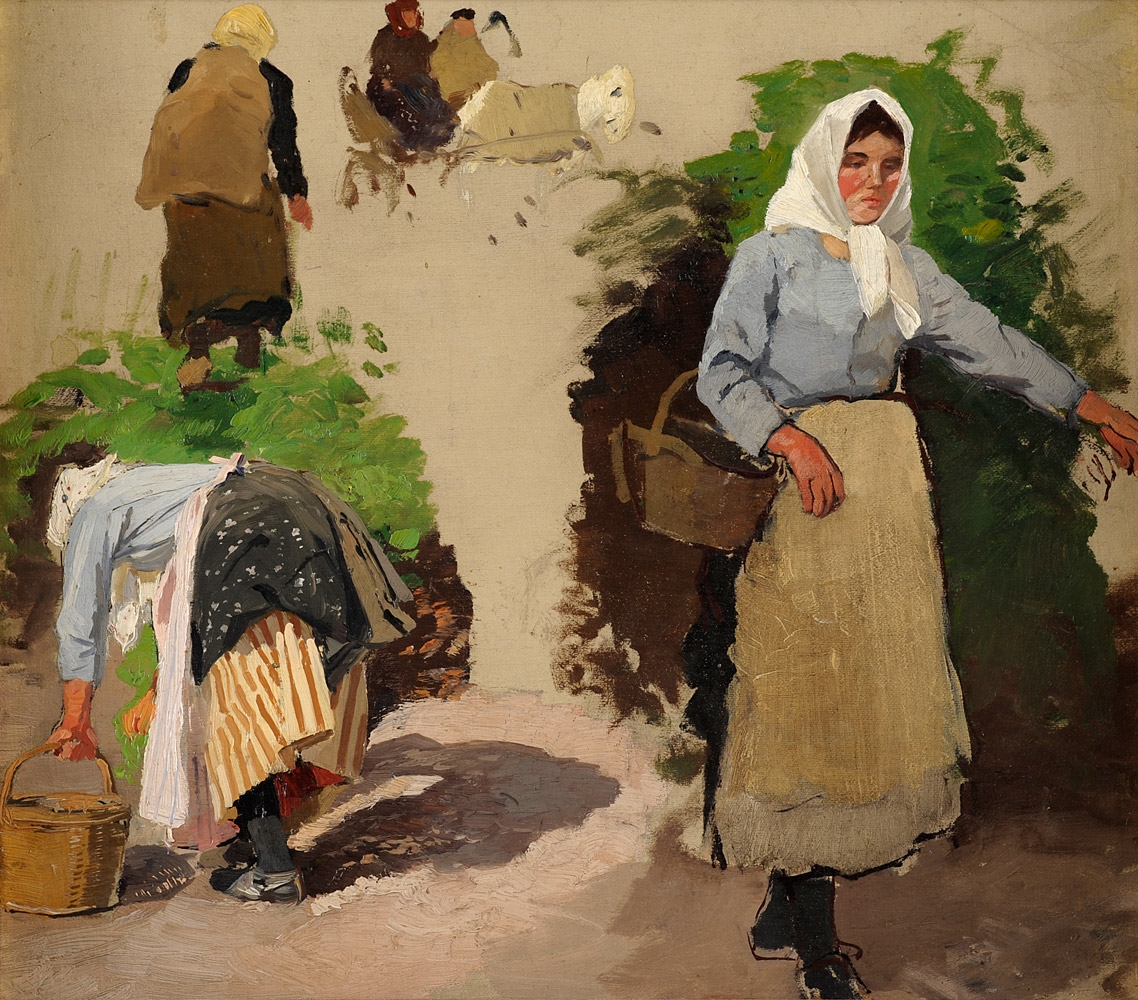This fine art painting features four distinct figures set against a predominantly brown background, each engaged in activities that evoke a sense of labor and pastoral life. On the right, a woman in a blue blouse and brown skirt, with a white bandana tied over her head, carries a basket on her right arm. She stands in front of a green bush, providing a stark contrast against the brown backdrop. To her left, another woman bends over as if to pick something up, gripping a basket in her left hand. She wears a blue blouse, white apron, and a layered skirt with colorful red and white stripes peeking out. Her head is also covered with a white scarf, and she stands in front of a green bush. Further behind her, a man carrying a large brown pack on his back walks away, blending into a less detailed greenish-brown scene. In the upper middle section of the painting, two figures, possibly riding on a horse, are rendered in brown tones, adding a distant, almost ethereal presence to the composition. This juxtaposition of figures engaged in various tasks, each with distinct attire yet unified by a common background, gives the painting a cohesive portrayal of rural life.